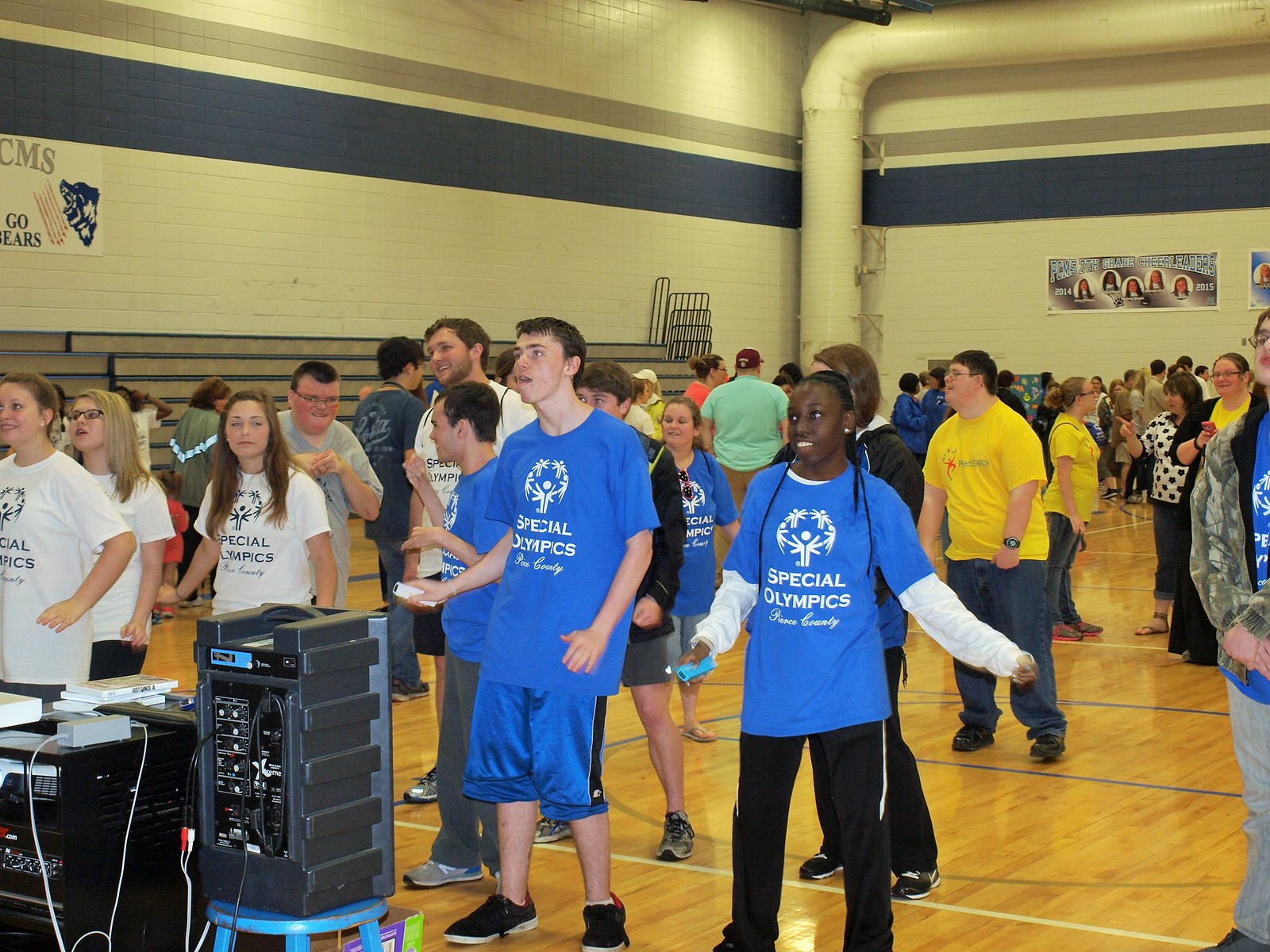In the photograph taken inside a gymnasium, likely at a high school or junior high, the setting is vibrant and engaging. The gym's walls feature a white background adorned with a large horizontal navy blue stripe and a gray stripe above it, extending across the width of the wall. Piping is visible emerging from the building in the background, adding to the architectural detail. On the gym’s polished hardwood floor, numerous students are gathered, creating a lively scene. They are dressed in a variety of colored shirts—blue, white, and yellow—each emblazoned with the words "Special Olympics," indicating that this is an event associated with the organization. The students, all smiling and facing the camera, exude happiness and excitement, capturing the joyful spirit of the Special Olympics event.